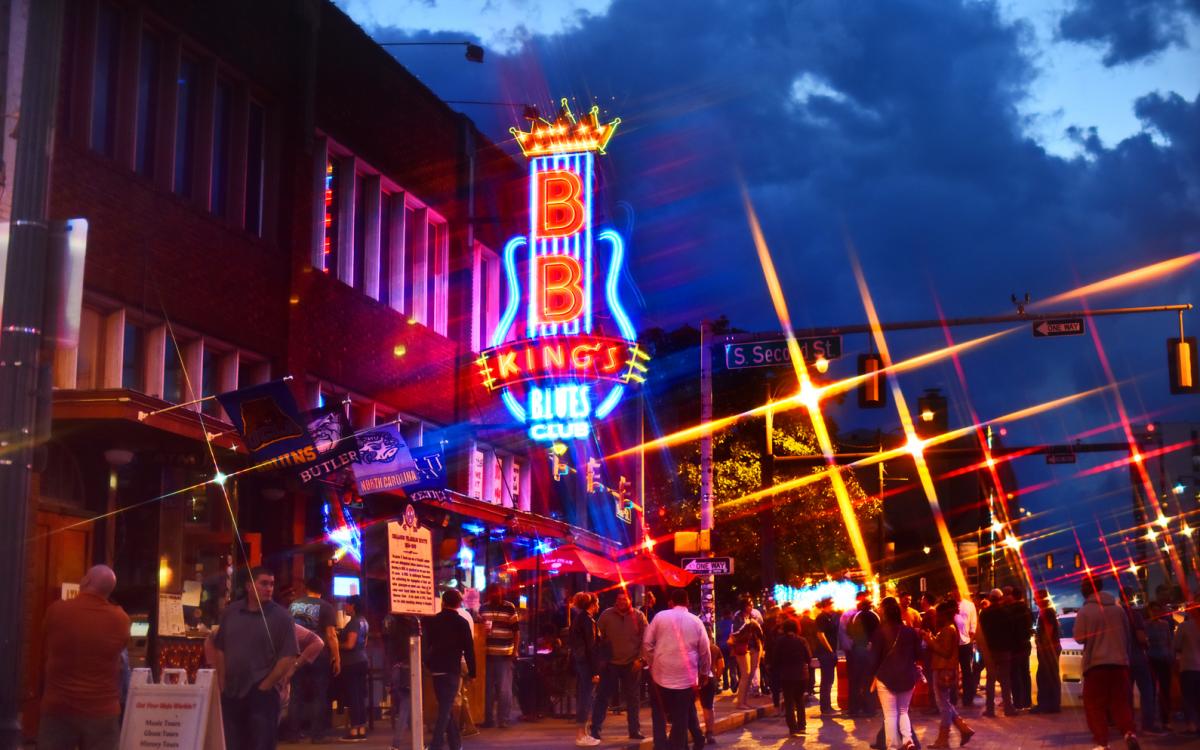The image captures a bustling street corner in the evening, likely Beale Street in Memphis or possibly Nashville, under a dark, cloudy sky. The scene is alive with brightly lit streetlights appearing as starbursts, creating an almost festive atmosphere. The focal point is B.B. King's Blues Club on the left side of the street. Its large, neon blue sign, shaped like a guitar with a crown on top, illuminates the area. An adjacent brown building stands behind the iconic sign. Adding to the vibrancy, a nearby traffic light flashes red, and there are several signs including one for South 2nd Street and a one-way sign on the light post. The street is crowded with people, many of whom are nicely dressed, possibly drawn by the lively aura of the club. Additionally, there are team flags hanging on the left side of the building, one stating "Butler North Carolina." The energetic hustle and bustle suggest it is a popular party spot, with numerous pedestrians walking on the sidewalk, seemingly eager to enter the club.